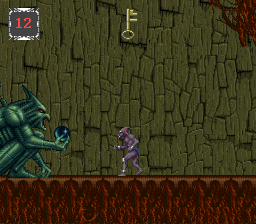This is a square picture depicting a simplistic 2D computer game. The bottom of the image features a brown strip resembling a floor or banner, clearly defining the base layer of the scene. The background is characterized by an interlocking, rocky texture with a greenish hue, giving it a rough, natural appearance. At the center of the image, a small gray creature is seen walking towards the left. Positioned on the lower left side of the scene is a menacing green monster with devilish features, including glowing red eyes and an outstretched hand, seemingly ready to intercept the creature. In the upper middle part of the image, a golden key floats, indicating an objective or collectible item. Additionally, the upper left corner contains a small black box displaying the number "12" in vivid red digits.